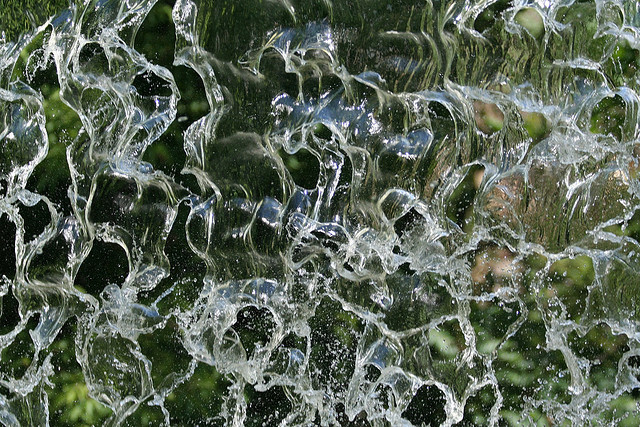This image depicts a fascinating, close-up view of water in mid-movement, seemingly frozen in time. The water, crystal clear and sparkling, splashes and swirls intricately, creating a captivating, almost surreal effect. The background is dominated by dark green hues, which are so deep they verge on black, suggesting a dense, swamp-like or forested area. This dark, green backdrop is slightly blurred, making it difficult to discern specific details but reinforcing a natural, leafy environment. The water appears to be in a state of dynamic suspension, with splashes and droplets forming sharp, translucent arcs and patterns, suggesting either a waterfall cascading down or a fountain spraying in various directions. The combination of the water's mid-air suspension and its interplay with the lush, shadowy background creates a visually striking and complex scene, evoking a sense of chaotic beauty and natural wonder.